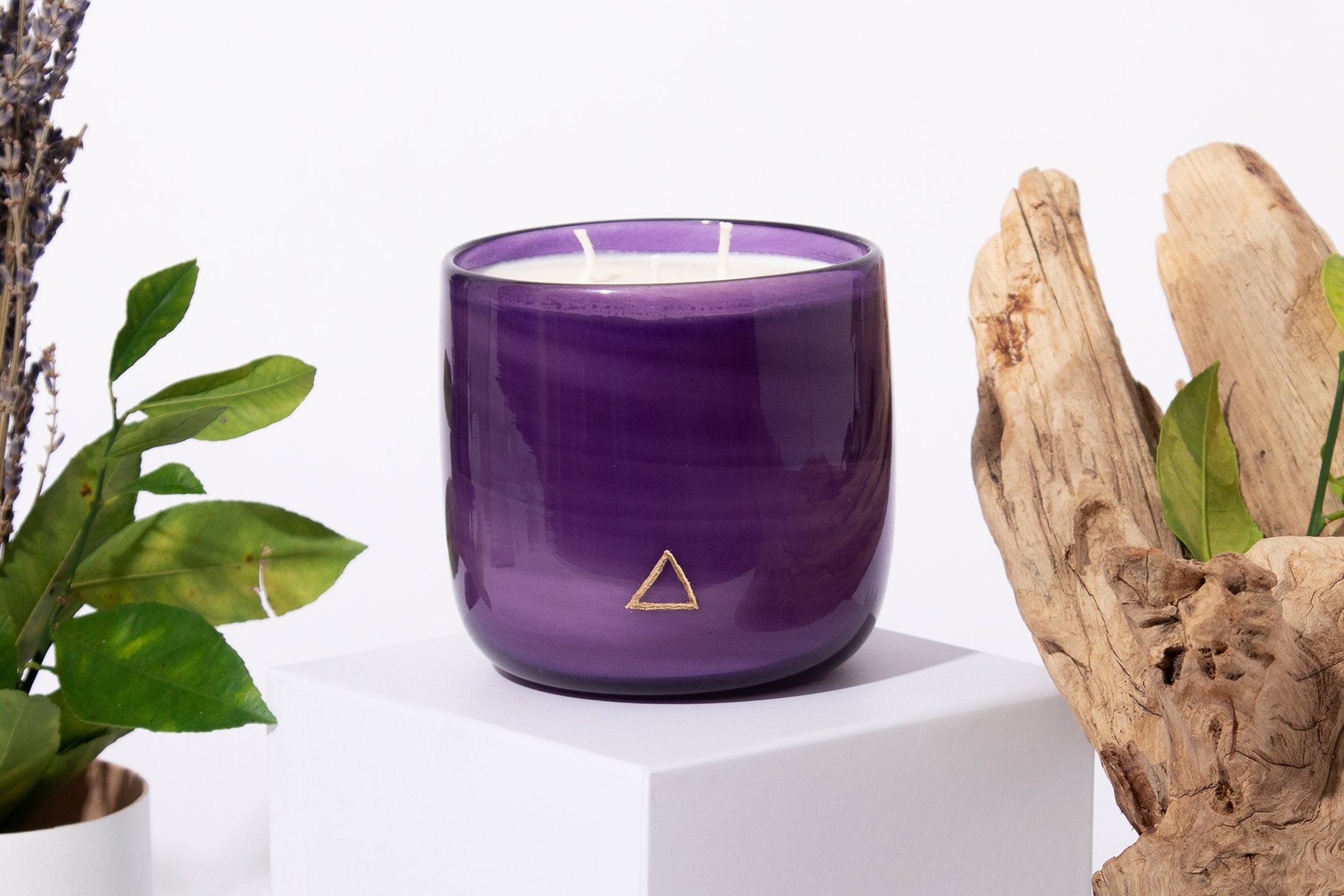The photograph depicts a professional-quality image centered around a purple candle encased in a glass jar, which features a gold triangle near its base. Inside the jar is white wax with two wicks. The candle is positioned on a white platform, likely a cube, casting a dark shadow. To the left of the candle, there is a white plant holder containing large green leaves, and to the right, there is a decorative piece of bark or a wooden figurine with some leaves inside. The background is a plain white wall, emphasizing the central elements of the image.